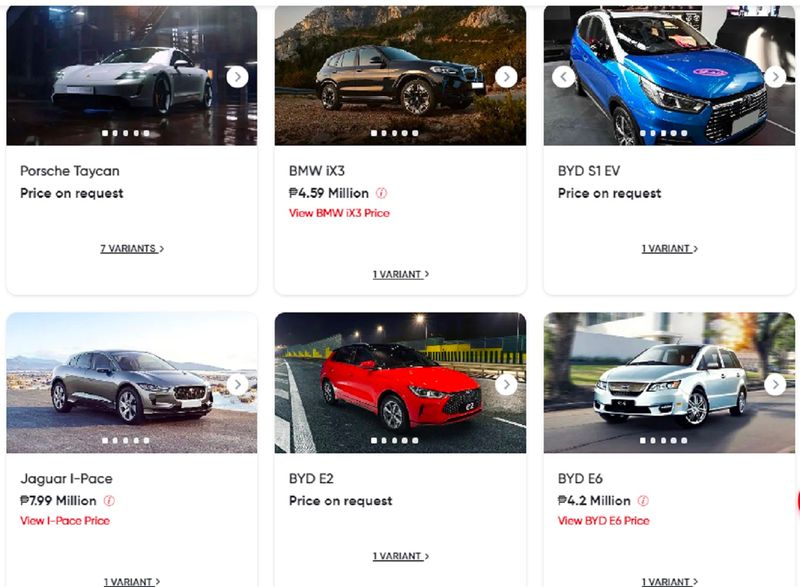The image appears to be a screenshot from a computer, displaying a grid of car images arranged in two rows, with three cars in each row. The cars are showcased in various settings, and each has a brief description beneath it.

**Top Row:**
1. **Gray Porsche**: Positioned in the upper-left corner, the gray Porsche is photographed on a showroom floor. The caption beneath it reads, "Porsche Taycan, price on request, seven variants."
2. **BMW**: Centrally located in the top row, this BMW is set against a mountainous backdrop. The description states, "BMW iX3, $4.59 million," followed by a link to view the BMW iX3 price and the note "one variant."
3. **Blue Car**: On the rightmost side of the top row, there is a blue car on a gray floor. Its caption says, "BYD S1 EV, price on request, one variant."

**Second Row:**
1. **Gray Jaguar**: Kicking off the second row on the left, a gray Jaguar is depicted outdoors with the sky as its background. The description below reads, "Jaguar I-Pace, $7.99 million," along with a link to view the Jaguar I-Pace price and the note "one variant."
2. **Red Car**: In the middle of the second row, this red car is shown on a black road. Its caption states, "BYD E2, price on request, one variant."
3. **Silver Car**: Completing the grid on the rightmost side, the silver car is displayed on a road. The description says, "BYD E6, $4.2 million," followed by a link to view the BYD E6 price and the note "one variant."

The layout of the image is orderly, providing clear visual and textual information about each car model.